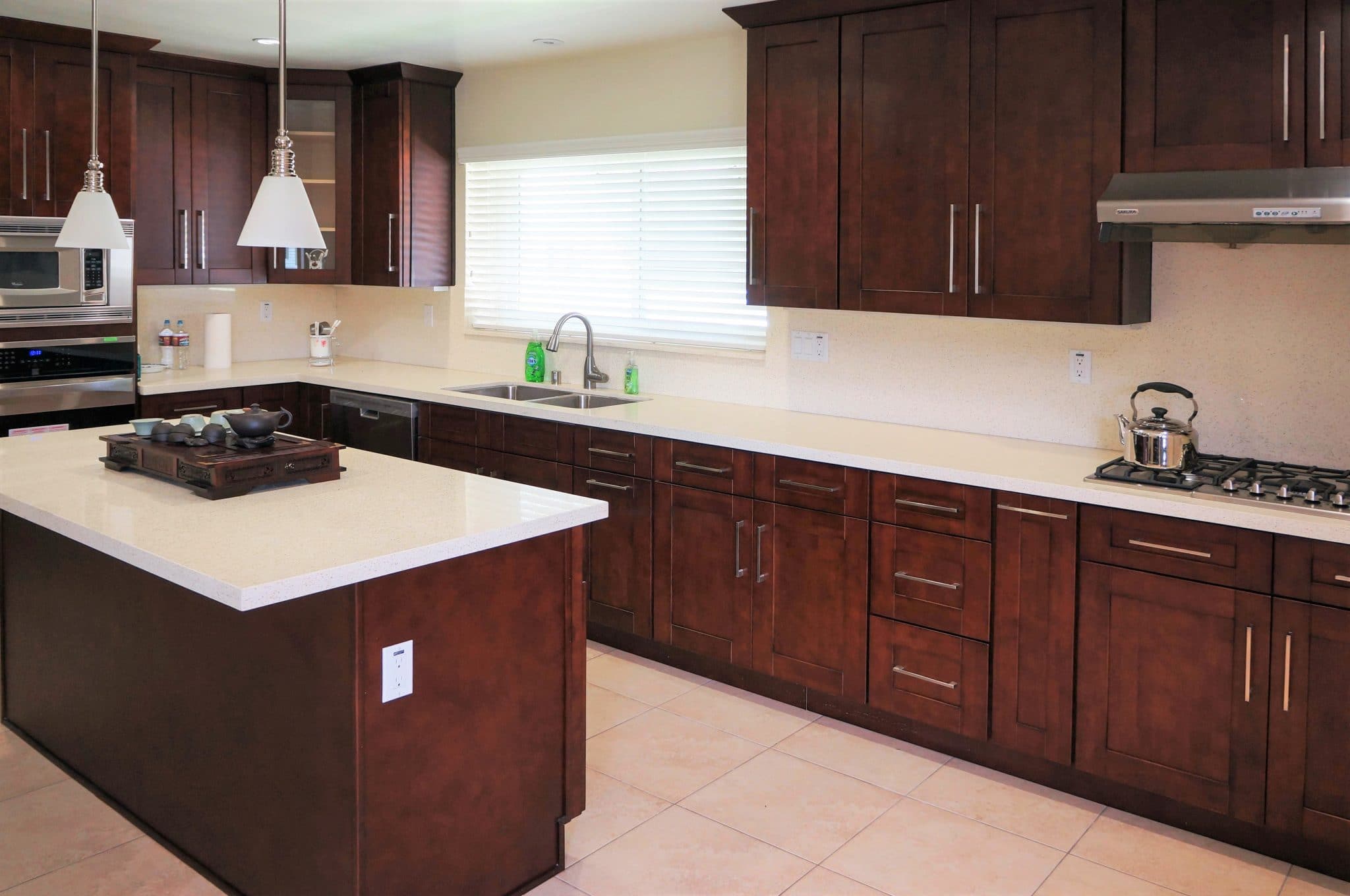This angled shot captures a sleek and modern kitchen, characterized by its clean lines and minimalistic design. The cabinetry, finished in a rich cherry wood or dark mahogany color, lines the kitchen and features silver bar handles, giving it a contemporary touch. The kitchen island, matching the cabinetry in color, stands centrally with a large white slate countertop, complemented by white stone counters that wrap around the kitchen. Above the island hang two white pendant lights, casting a warm glow over a small wooden tray that holds a tea set.

The kitchen walls are painted a subtle ecru, a yellowish-white hue that brightens the space. A large rectangular window with closed white blinds sits above the stainless steel sink, which is accompanied by two green dish detergent bottles. To the right, the stove and oven combo with a microwave above them provide ample cooking facilities, and a metal teapot sits ready on the stovetop. The range hood above the stove is sleek and silver, fitting seamlessly into the modern design.  Additionally, there are two electrical outlets on the island, adding functionality to the stylish space. The overall feel is one of pristine, unused openness, suggesting that the house might be newly listed for sale.